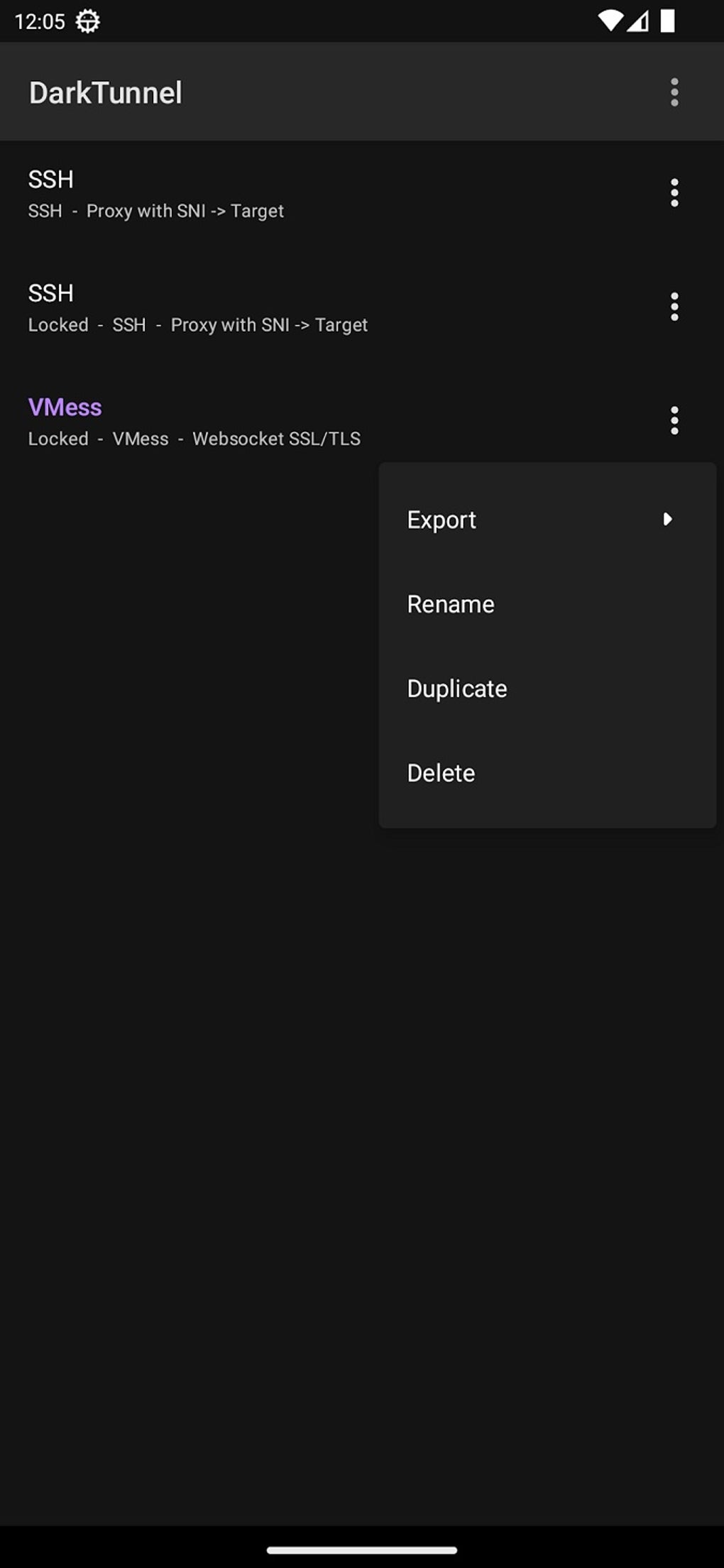A detailed screenshot of a back-end settings page in an app with a dark mode theme. The background is black with white or light gray text. At the top of the interface, a gray bar spans across the screen, displaying "Dark Tunnel" on the left side. On the right side of this bar, there is a three-dot icon for accessing additional options. Below this bar, there are three sections, each containing relevant descriptions and settings, accompanied by a three-dot icon on the right for further actions.

1. **SSH**: The section labeled "SSH" has the description "SSH proxy with SNI arrow to target" below it.
2. **SSH Locked**: This section is marked as "SSH locked" and includes the description "SSH proxy with SNI arrow to target".
3. **vMess**: This section is highlighted in purple and labeled as "vMess" with the description "Locked vMess WebSocket SSL/TLS".

Additionally, a context menu appears in the bottom-right corner of the screenshot, offering options to "Export," "Rename," "Duplicate," and "Delete" settings.